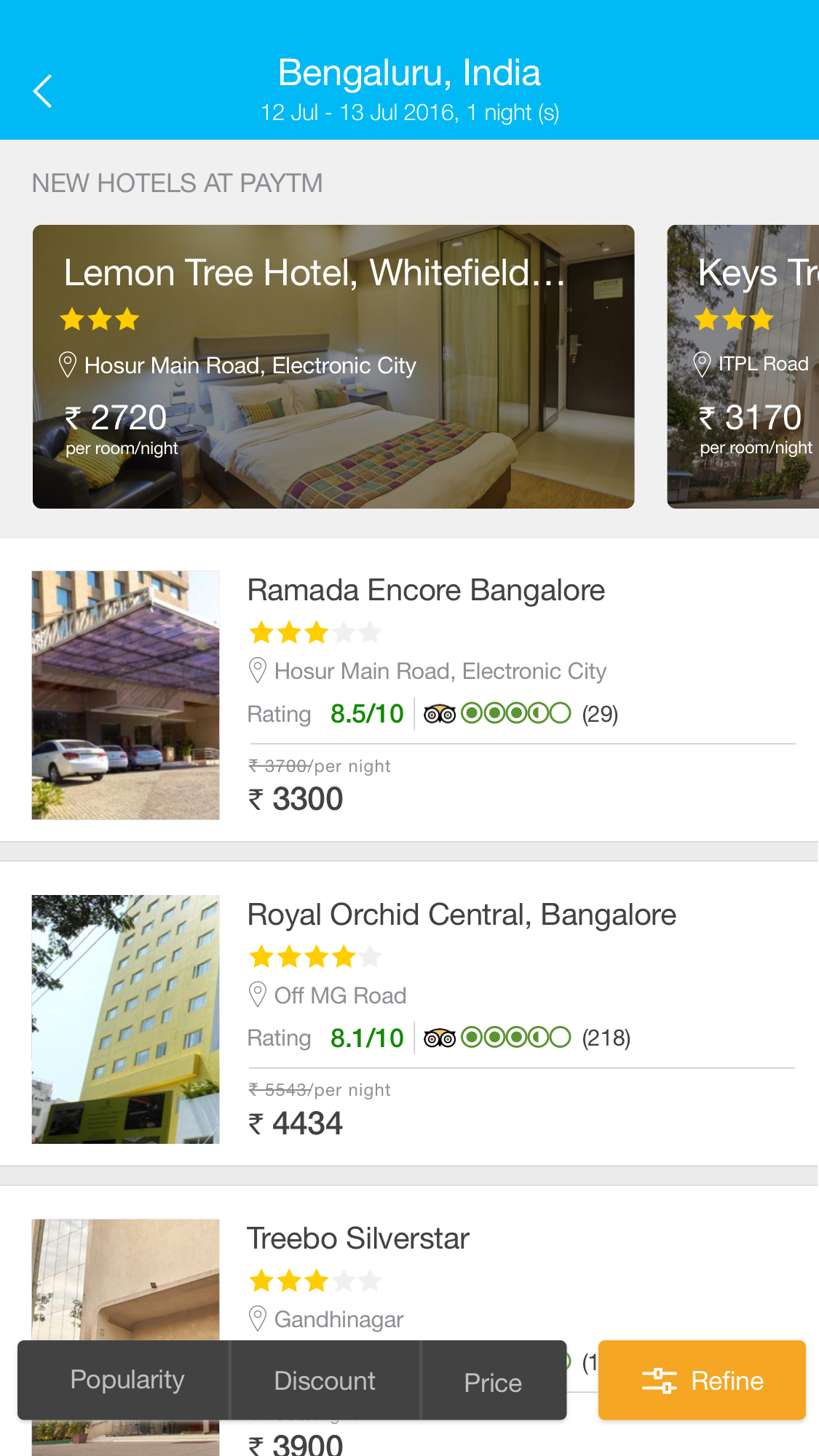In the image, we see a screenshot of a smartphone displaying a hotel booking page on the TripAdvisor app, identified by its distinctive logo. The search parameters are set for Bengaluru (Bangalore), India, with a one-night stay from July 12th to July 13th, 2016. 

The screen lists several hotels along with their nightly rates in Indian Rupees:
1. **Lemon Tree Hotel, Whitefield** - ₹2,220 per night.
2. **Ramada Encore Bangalore** - ₹3,300 per night.
3. **Royal Orchid Central Bangalore** - ₹4,434 per night, featuring a four-star rating.
4. **Tribo Silver Star** - ₹3,900 per night.

At the bottom of the screen, there are filter options available to refine the search by price, discounts, and popularity. The listed hotels come with various star ratings, providing users with options for different budget ranges and preferences.